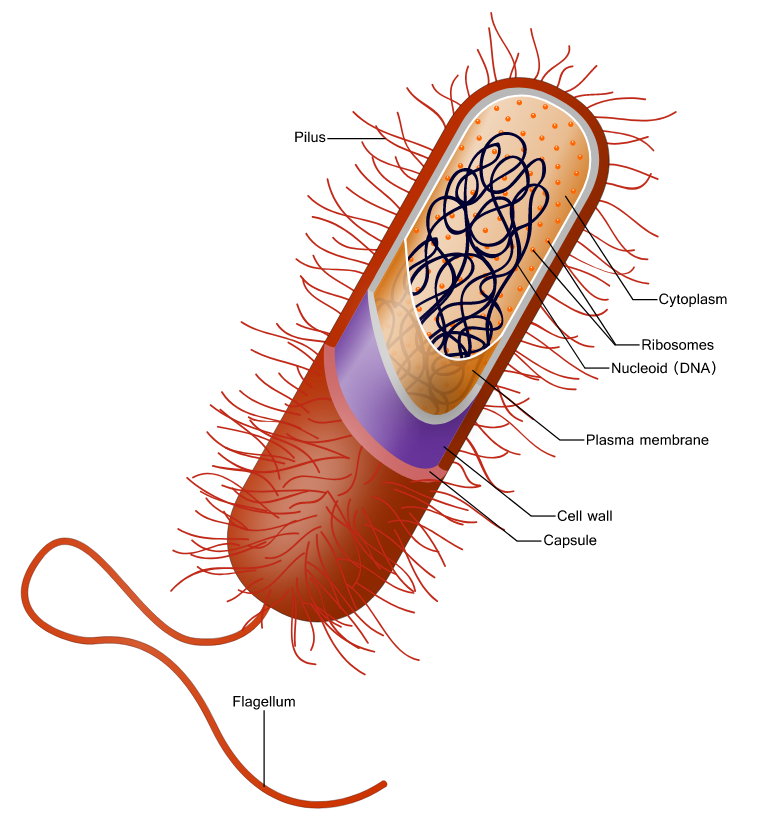The image is a detailed, artistic representation of a virus against a stark white background. The virus appears as an elongated, spherical entity predominantly colored in shades of pink, red, and orange. The outer surface of the virus is covered with hair-like follicles labeled as "Pilus." Further examination reveals a segmentation within the virus: a purple section at the top and an orange section surrounding a series of orange dots identified as ribosomes and black, stringy lines labeled as nucleoid DNA. These segments are encased in cytoplasm and enveloped by layers of the plasma membrane, cell wall, and capsule. On the outside, each component is meticulously labeled in black font: pilus, cytoplasm, ribosomes, nucleoid DNA, plasma membrane, cell wall, and capsule. At the bottom of the virus, a long, swirling tail designated as the flagellum extends outwards, also colored in orange.